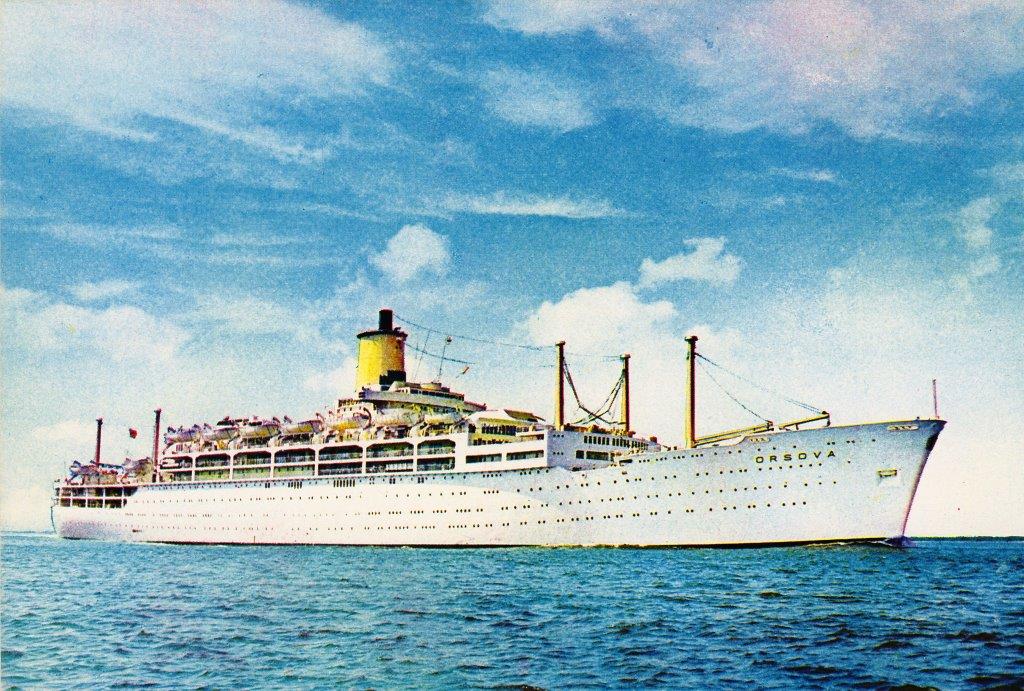The image shows a long, white cruise ship named "Orsova" prominently displayed on its side, sailing in a very blue, clear sea. The Orsova is almost the entire length of the frame, emphasizing its massive scale. The top section of the ship includes various structures painted yellow, including a large chimney with several strings attached, reminiscent of a vintage steamer. The sky above is light blue with some clouds, adding a serene backdrop. Numerous windows line the side of the ship, suggesting it is carrying many passengers embarking on a voyage. The water exhibits ripples and waves, contributing to the dynamic scene, and the entire composition resembles a detailed painting.